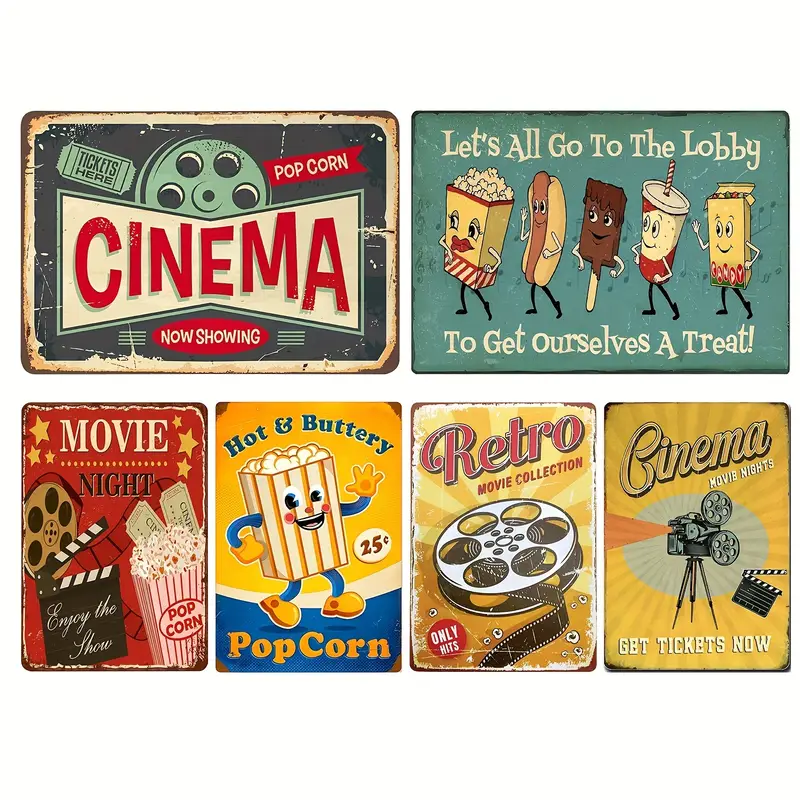The image is a vibrant, well-lit collage featuring retro cinema posters. At the top left, a horizontal poster reads "Tickets Here," "Popcorn," and "Cinema," set above a banner declaring "Now Showing," accompanied by a movie reel and a ticket image. The top right poster, also horizontal with a turquoise background, cheerfully suggests, "Let's All Go to the Lobby to Get Ourselves a Treat," portraying animated food items— a popcorn bag, a hot dog, a chocolate fudgesicle, a soda cup with a straw, and a candy box— moving to the left.

The bottom section consists of four vertical posters. The bottom left poster announces "Movie Night" with the directive "Enjoy the Show," featuring a film reel, a director's clapperboard, a popcorn box, and a pair of tickets. Adjacent to it is a vintage-style poster with an anthropomorphic popcorn box, proclaiming "Hot and Buttery Popcorn 25 cents." The next poster highlights a "Retro Movie Collection," adorned with a film reel and the promise of "Only Hits." Lastly, the bottom right poster urges viewers to "Get Tickets Now" for "Cinema Movie Nights," depicted with a classic movie camera and another director's clapperboard. Each poster is distinct and vividly clear, thanks to the bright lighting enhancing the nostalgic theme.